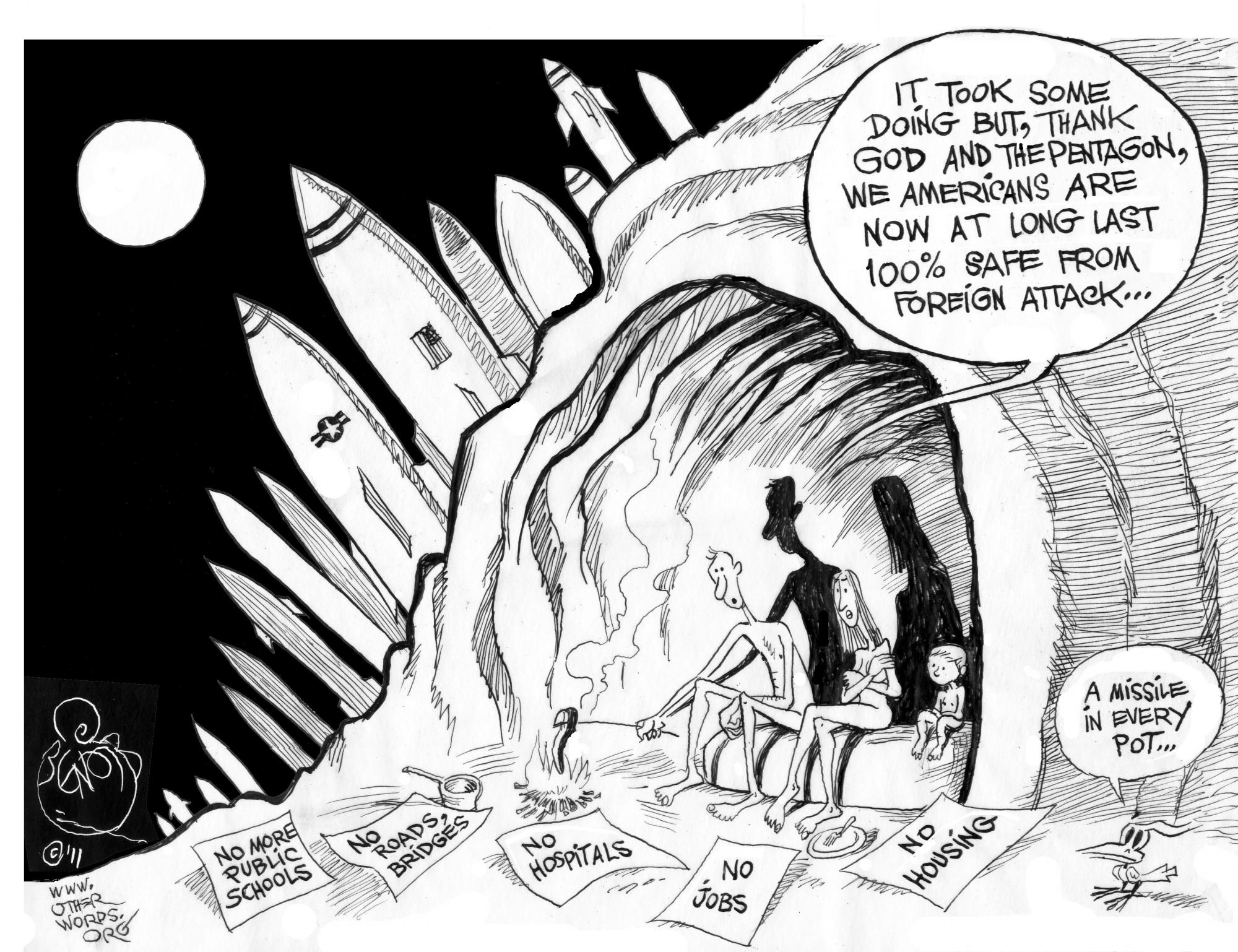In this black and white political cartoon, a man, woman, and child sit completely nude inside a dark, shaded cave, their expressions depicting fear and cold. The man is cooking a shoe over a small fire, casting ominous shadows on the cave walls behind them. The details of their plight are emphasized by numerous pieces of paper scattered on the ground, each marked with stark phrases such as "no more public schools," "no roads, bridges," "no hospitals," "no jobs," and "no housing." A small bird on the right side adds a bleak touch with a sign that says, "a missile in every pot." The scene is further intensified by an array of nuclear missiles poised for launch outside the cave. Above, a thought bubble reads, "It took some doing, but thank God in the Pentagon we Americans are now at long last 100% safe from foreign attack." This cartoon delivers a powerful critique on the excessive defense spending at the cost of basic public services and living conditions, humorously yet grimly illustrated by the family’s dire circumstances.